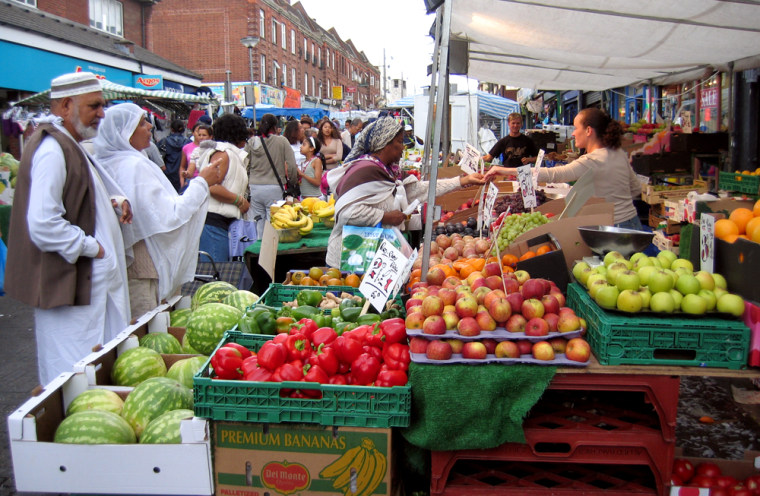The photograph depicts a bustling farmer's market, likely situated in a downtown Middle Eastern area, visible through its vibrant scene and cultural elements. Centered in the frame is a prominent stand showcasing a rich array of produce. The display spans five levels, featuring watermelons, red and green bell peppers, red and green apples, oranges, tomatoes in white boxes, and plums. Notably, there is a crate labeled "premium bananas" supporting a group of red bell peppers, while red apples rest atop a blue surface.

People swarm the market, engaged in various activities. One woman in Middle Eastern attire, identifiable by her white robe and head covering, is exchanging money with a vendor. Behind the stand, two workers attend to customers. In the left foreground, two more individuals in traditional Middle Eastern garments survey the produce.

The setting extends beyond the market, revealing a lively street with a mix of architectural elements. A large red brick building and adjacent structures with blue awnings and vividly colored signs add to the dynamic backdrop. Above the market, white cloth awnings provide shade, while other parts of the market remain exposed to the open street. This captivating scene is framed horizontally, capturing the essence of daily life and commerce in a vibrant community space.